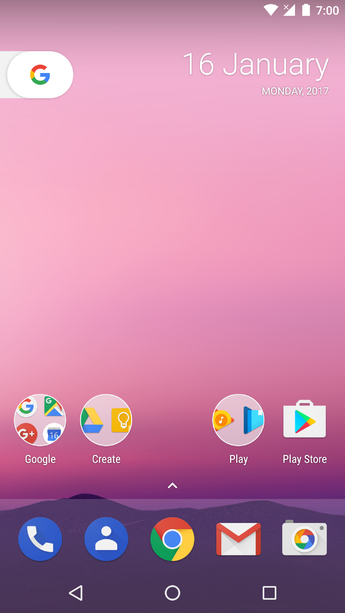The image showcases a smartphone interface with the following details:

- At the top of the screen, the status bar displays a full Wi-Fi signal, full battery icon, and the time set at 7:00. The date is January 16, 2017, which is a Monday.
- The background features a gradient of colors, transitioning from pink at the top to purple at the bottom.
- On the home screen, the bottom left corner displays app icons for G, Maps, Google+, Calendar, and Google Create.
- There is text that reads "We Drive" alongside a yellow circle and square, followed by a set of orange and blue triangles.
- The center of the screen shows icons for the Play Store, a blue circle with a person symbol, Google Chrome, Gmail, and the camera.
- A Google Chrome logo appears, characterized by a circle containing a sideways triangle.
- The center circle is surrounded by a square icon and a wavy, hill-like pattern in the background, blending red and pink hues.
- Monday, 2017, is also noted as part of the background design.

The overall impression is of a vibrant and colorful smartphone display with a variety of app icons and background elements blending seamlessly.